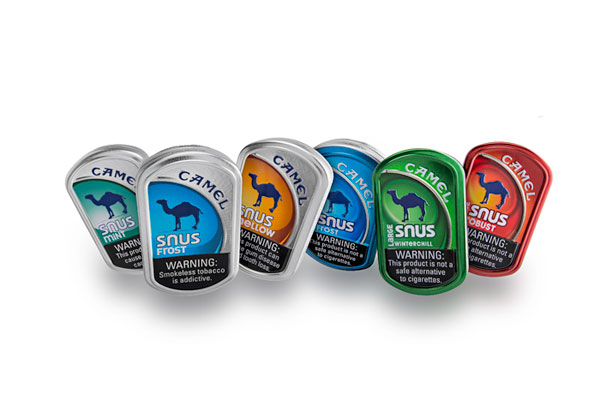The image features a horizontal row of six Camel Snus cans aligned centrally against a stark white background, giving it a stock image or advertisement feel. From left to right, the cans are arranged as follows: the first can is Mint with a teal color, the second is Frost in an icy blue shade, the third, partially visible, appears to be Mellow (formerly identified as Yellow) in a cross between orange and yellow, the fourth repeats Frost in a similar blue hue, the fifth is Winter Chill in a green color, and the last can is Robust, predominantly red with hints of orange. Each can is topped with a chrome-colored lid, except for the last three, which are fully colored. A consistent feature on all cans is a prominent blue camel logo in the center and a black warning label at the bottom that reads, "Warning: smokeless tobacco is addictive." The cans' varying angles cast shadows, adding depth to the otherwise clean and minimalistic composition.